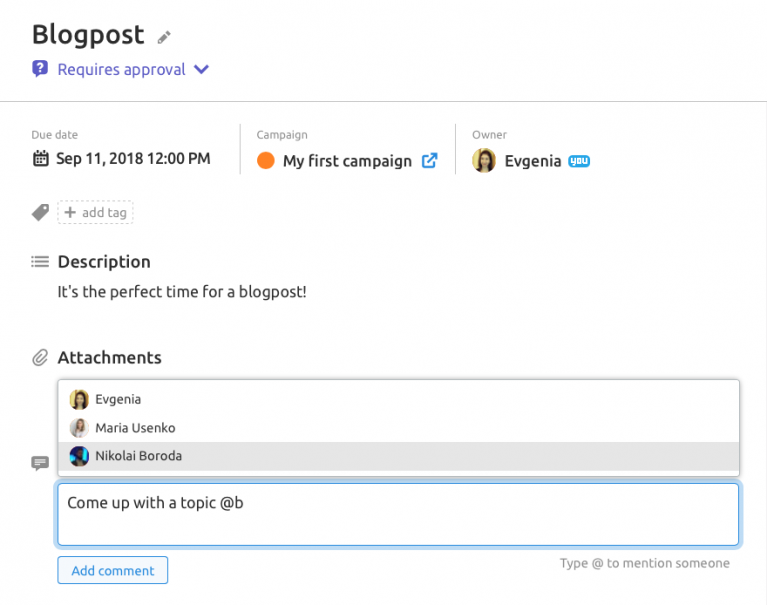Caption: 

This image depicts a blog post awaiting approval, with a due date set for September 11, 2018, at 12 p.m. The blog post is part of a campaign titled "My First Campaign," and it is owned by Benji. The tags include a description stating, "The perfect time for a blog post!" The interface features several functionalities: attachments for adding various documents or relevant files, an option to mention specific individuals using the "@" symbol for targeted communication, a question mark icon at the top for accessing help or additional information, and an edit pencil icon for making modifications to the content. Users associated with this campaign include Benji, Maria Yasinko, and Nikolai Borado. There is a note prompting, "Come up with a topic at B," possibly indicating further instructions or assignments.